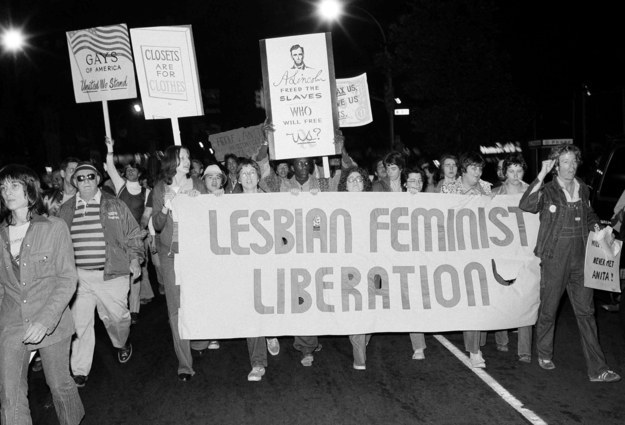This horizontally aligned rectangular black and white photo, taken at nighttime, captures a vibrant parade or protest. The sky at the top of the image is solid black, dotted by a couple of blurry spotlights that resemble stars, located in the upper middle and upper left areas. Marching down a street, the foreground is dominated by a large, white rectangular banner bearing the bold, all-caps inscription "LESBIAN FEMINIST LIBERATION." Behind this banner, various additional signs are being held aloft: one reads "GAYS OF AMERICA UNITED WE STAND," another states "CLOSETS ARE FOR CLOTHES," and a third sign, featuring an image of Abraham Lincoln, declares "ABRAHAM FREED THE SLAVES WHO WILL FREE US." 

In the lower right corner, the street’s white stripe is visible, grounding the scene in its urban setting. Among the diverse crowd—comprising people of different nationalities, shapes, sizes, and ages—stands a woman on the right, carrying a personalized sign with the word "Anita" on it. Despite the night's darkness, there's an air of unity and happiness among the marchers, illuminated gently by the streetlights.